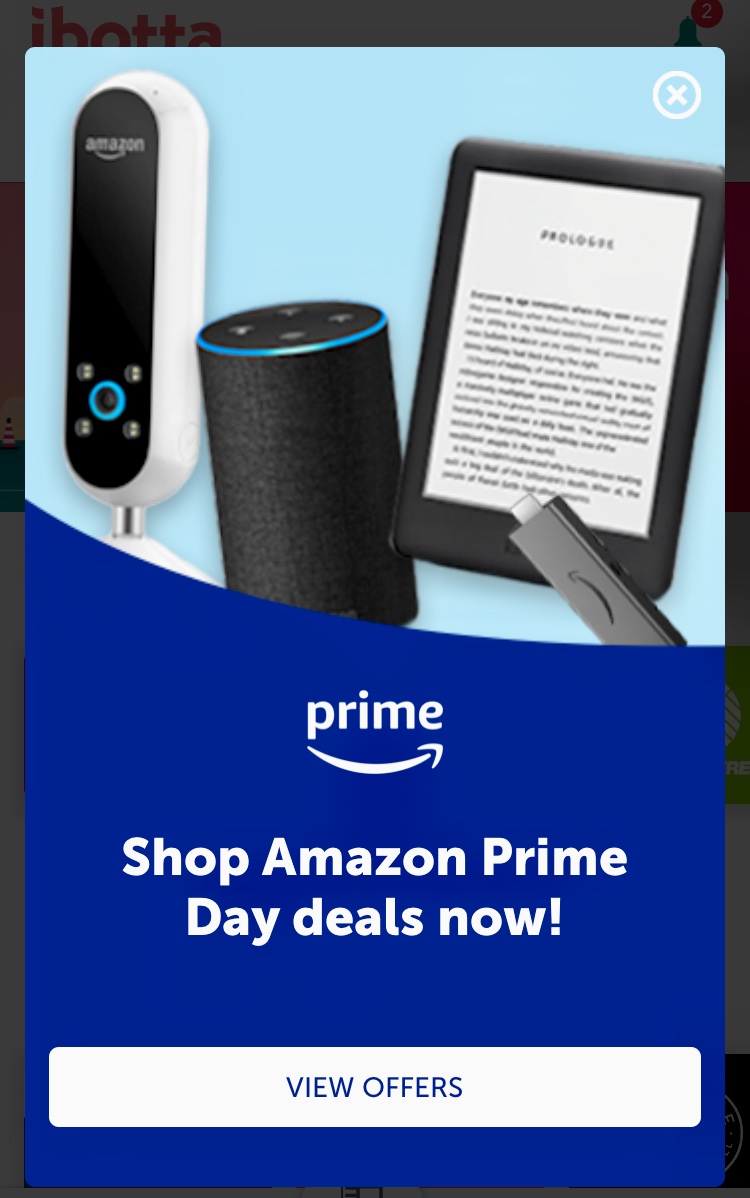The advertisement promotes the exclusive Amazon Prime Day shopping event for Amazon Prime members. It prominently features three of Amazon's flagship products: the Amazon Echo device, a Fire Stick, and a Kindle e-reader, showcasing the variety of tech deals available during Prime Day. The visual design includes a sharp blue background, which not only grabs attention but also creates a sense of urgency. Central to the ad is a bold, white text that reads "Shop Amazon Prime Day Deals Now!" encouraging immediate action. Below this, a large button with white text that says "View Offers" directs users to the Prime Day deals, emphasizing the call to action.